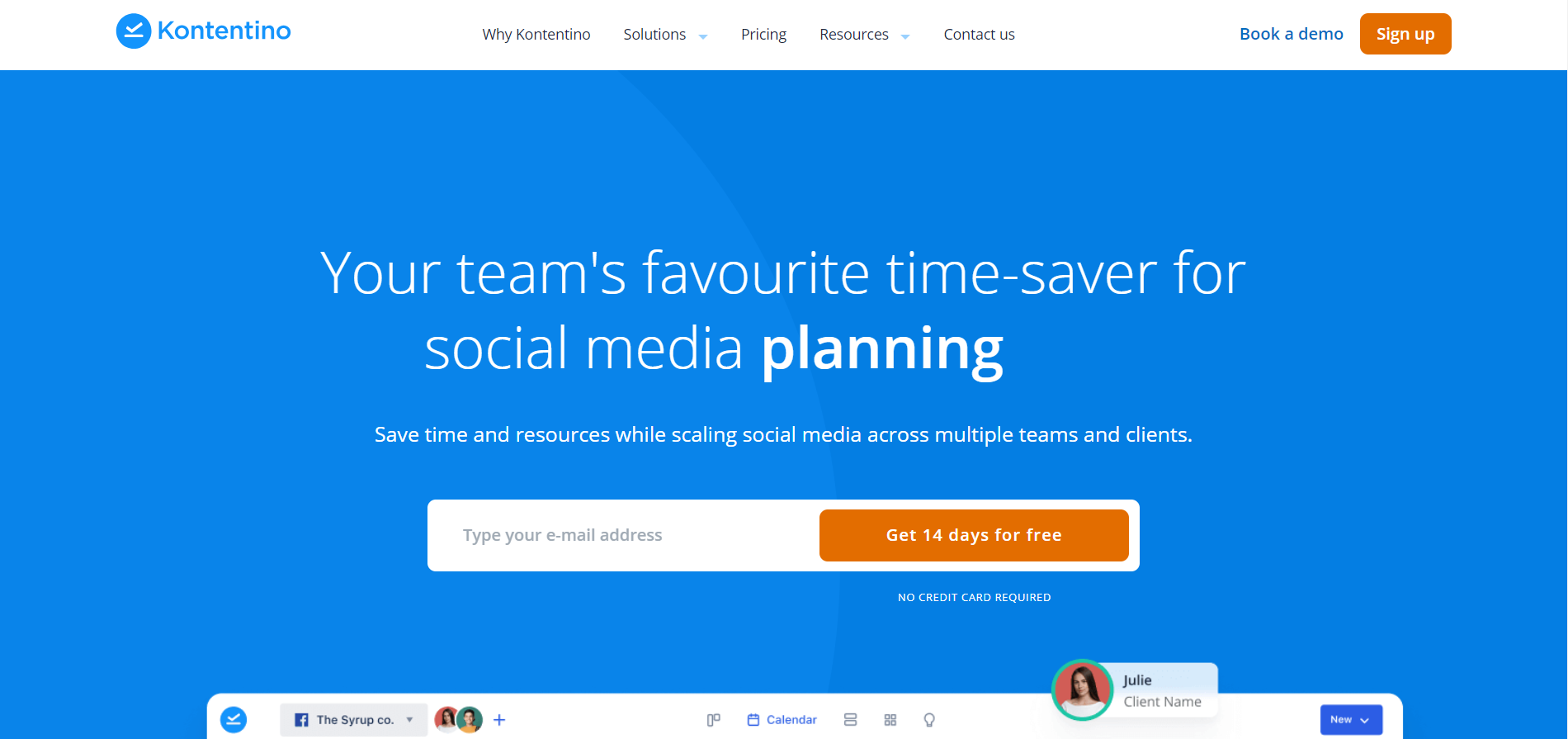This image showcases a well-organized website homepage layout, designed with a clean and professional aesthetic. At the top of the page, a white navigation bar prominently displays the logo "Contentino," accompanied by a small blue circle containing a white check mark. The navigation menu includes links like "Why Contentino," "Solutions," "Pricing," "Resources," "Contact Us," and a call-to-action button that reads "Book a Demo," all organized neatly to enhance user experience. On the far right of this bar, there is a noticeable red "Sign Up" button.

The central background is a visually pleasing blue, overlaid with the headline "Your Team's Favorite Time Saver for Social Media Planning." This is followed by supportive text: "Save time and resources while scaling social media across multiple teams and clients." Below this is an interactive section featuring a prominent search box inviting users to "Type your email address," paired with a red button labeled "Get 14 days for free," encouraging trial engagement. A small, slightly unreadable white line appears underneath this section, serving as a subtle separator.

Towards the bottom of the image is a series of white boxes. Among these elements is a small red circle featuring a white check mark and an underline, alongside familiar social media icons including the Facebook symbol. There are also two small profile pictures and a search box icon, indicative of social media management tools. Additionally, the calendar icon and tabs indicate scheduling functionalities. Notably, there is a small blue circle with a profile image of a woman labeled "Julie," along with a blue button that appears to be an interactive element, perhaps labeled "You."